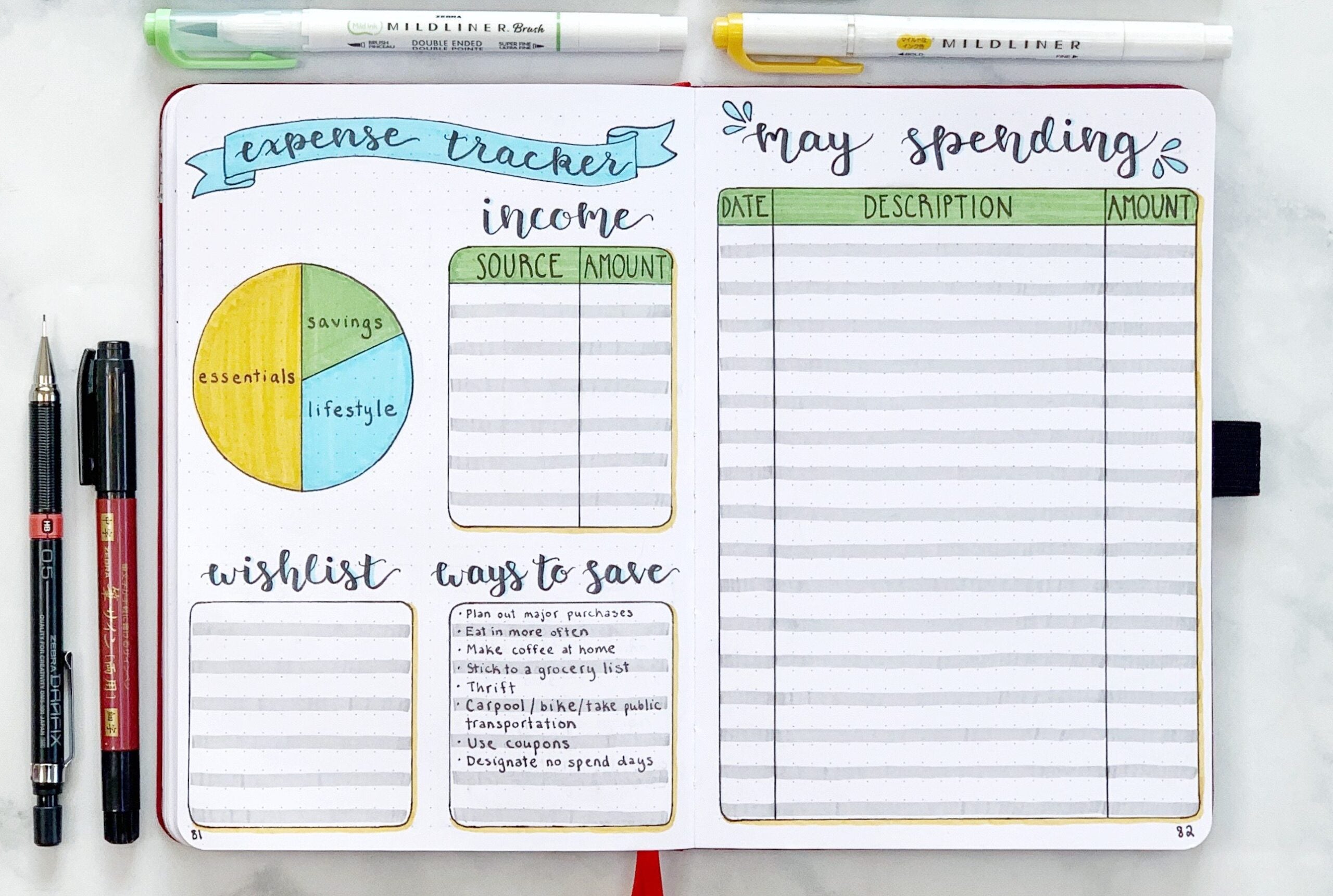The image showcases an open notebook with light dot grid pages, lying on a white marble surface. The notebook is horizontally rectangular with neatly rounded corners. At the top of each page, various organizational tools and diagrams have been meticulously sketched out.

On the left page, a blue banner labeled "Expense Tracker" is written in black cursive handwriting. Below this banner, a pie chart divides the expenses into three categories: Essentials, Savings, and Lifestyle. The essentials take up half the chart, while savings and lifestyle constitute roughly a third and a quarter respectively. Underneath, there are tables for tracking Income and Sources, a Wishlist with blank spaces for items, and a section titled "Ways to Save." This section offers practical tips such as planning major purchases, eating in more often, making coffee at home, sticking to a grocery list, thrifting, carpooling, biking, public transportation, using coupons, and designating no-spend days.

The right page continues the financial planning theme, starting with a heading "May Spending" adorned with small blue droplets. It includes a table with columns labeled Date, Description, and Amount, designed for users to log their expenditure details.

Two white markers, identified as Mildliners, are placed at the top center of the notebook, one with a light blue tip and the other with a yellow tip. Additionally, on the left side of the open notebook lie a black pen and a mechanical pencil, each accented with dark red details. This thoughtfully arranged scene is geared towards meticulous financial planning, presented in a visually appealing manner.